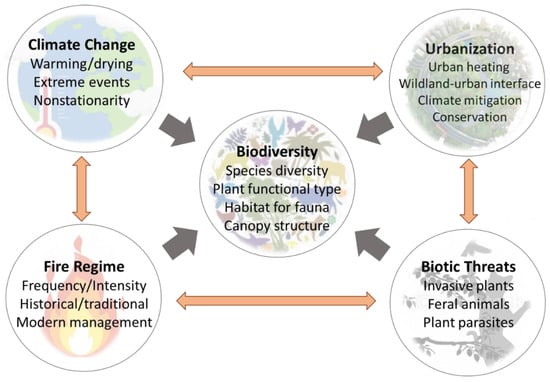This detailed diagram, set against a white background without a border, features five interconnected circles with different themes. At the upper left, the bolded text "Climate Change" is emphasized, with subpoints including "warming/drying," "extreme events," and "non-stationarity." From here, a two-way orange arrow connects to the upper right circle labeled "Urbanization," which highlights "urban heating," "wildland-urban interface," and "climate mitigation/conservation."

Another two-way orange arrow travels downward to the lower right circle, marked "Biotic Threats," mentioning "invasive plants," "feral animals," and "plant parasites." Extending leftward, another arrow links this circle to the lower left one called "Fire Regime," detailing "frequency/intensity" and "historical/traditional modern management."

All these outer circles have thick, short gray arrows converging on the central circle, which is titled "Biodiversity" in bold, with points about "species diversity," "plant functional type," "habitat for fauna," and "canopy structure." Together, these elements illustrate a complex network where climate change, urbanization, biotic threats, and fire regimes are interdependent and collectively impact biodiversity. A small paragraph is included, elaborating on the interactions and the cyclical nature of these themes.